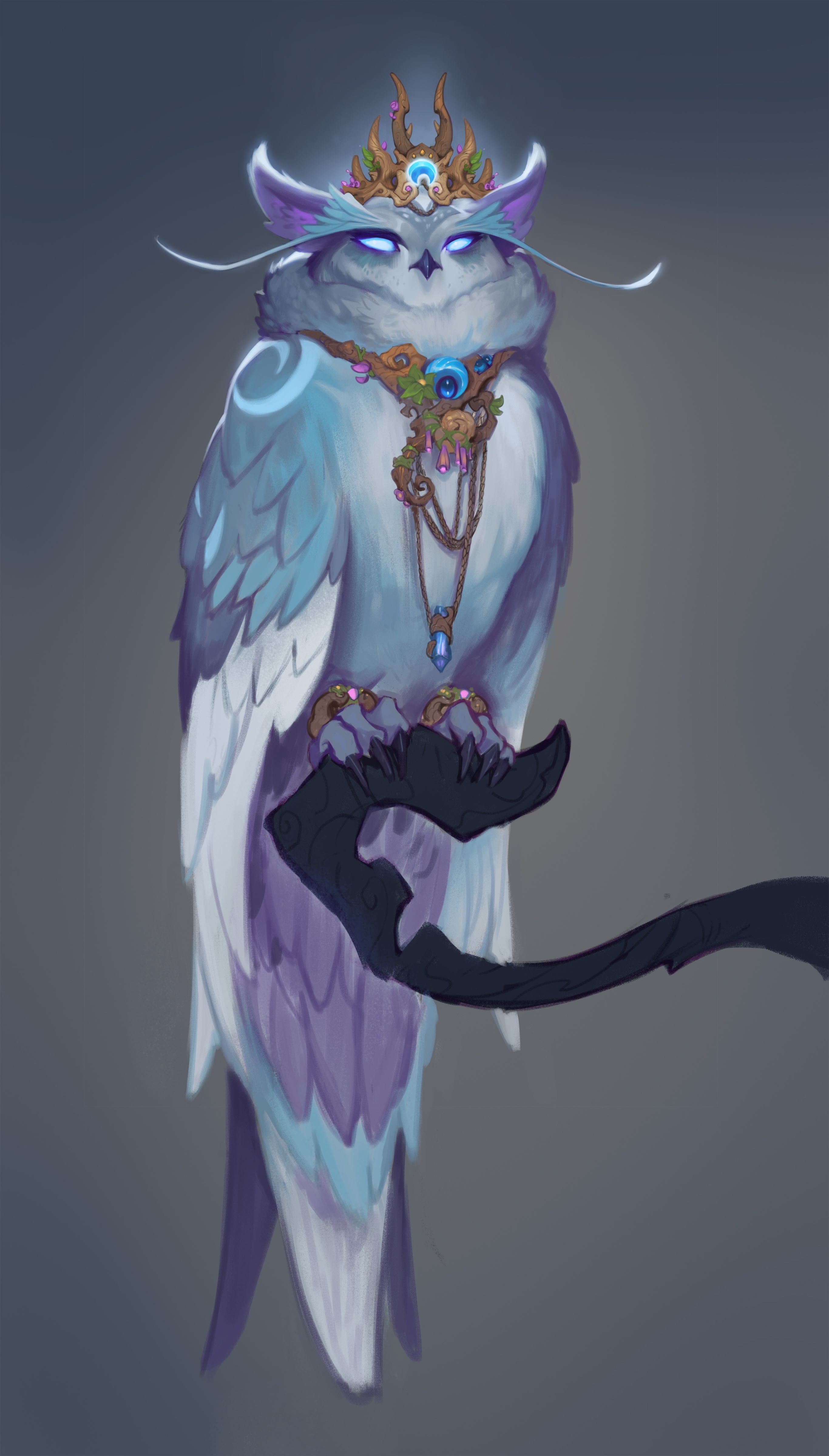The image depicts a fantastical creature, a hybrid of an owl and a cat, perched on the tip of a twisted, staff-like branch. The creature has a distinctive and majestic appearance, characterized by its elaborate plumage and royal accessories. Its feathers are primarily a blend of teal, blue, gray, white, and purple, with purple plumes transitioning to white at the tips. The wings, folded by its sides, showcase a gradient from dark blue on top to white at the bottom.

The owl-cat hybrid has a striking face that combines feline and avian features, with light blue, almost glowing eyes that give it a serious and somewhat eerie expression. Its small black beak and whiskers-like features on its eyebrows enhance its unique appearance, while its pointed cat ears frame its head. Atop its head rests a brown crown, adorned with stick-like elements and fiery details, complemented by accents of green and purple.

The creature also wears an ornate necklace, centered around a large blue orb, encircled by two smaller, duller orbs, and a chain with a light blue gemstone hanging down. Its talons, firmly gripping the dark branch, have three claws on each foot, each encircled by a dark brown ring with a pink gem at the center.

The background of the image is stark, composed of white and dark gray tones, which highlight the vibrant colors and intricate details of the owl-cat creature, making it the focal point of this enchanting artwork.